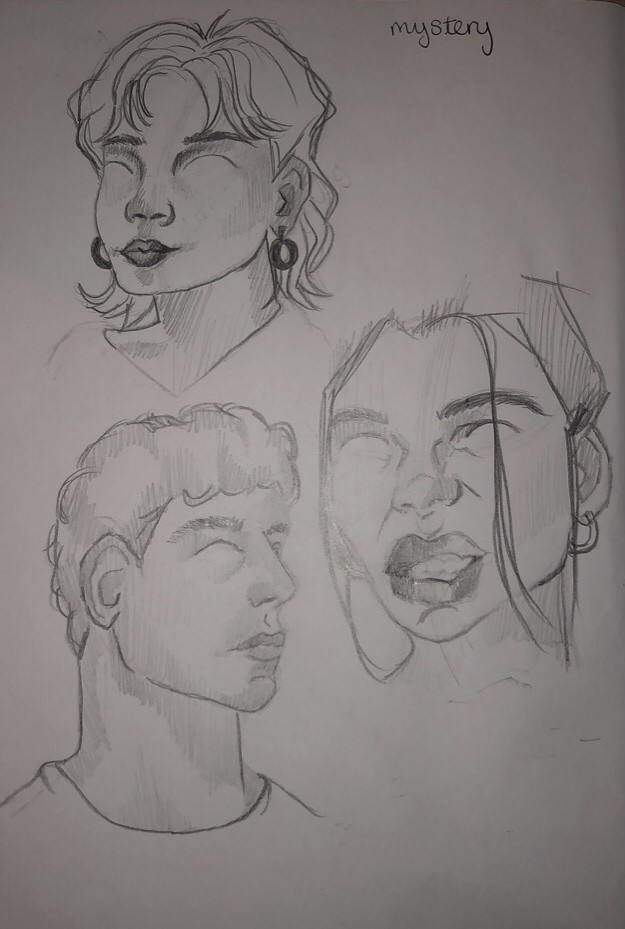This illustration depicts a detailed pencil drawing on a rectangular, white piece of paper. The word "mystery" is inscribed in small font near the top right corner. The paper showcases three finely shaded portraits.

At the top left is a woman with shoulder-length hair that extends to the back and short bangs. Her eyes are closed, displaying her eyebrows, and her dark lipstick emphasizes her pursed lips. She is adorned with hanging hoop earrings.

In the middle right section, there is another portrait, which might depict the same woman but from a different angle. Here, her hairstyle varies slightly, with a lock of hair falling on the left side of her face and more hair covering the right side. Her lips are parted, revealing her teeth, and she wears distinctive hoop earrings that appear to be either white or gold.

At the bottom left is a young man with curly, short hair ending at the top of his neck. His eyes are also closed, and he is facing towards the right. He appears to be wearing a t-shirt.

The artist's skillful shading brings depth to each portrait, enhancing the enigmatic quality suggested by the word "mystery" prominently featured on the paper.